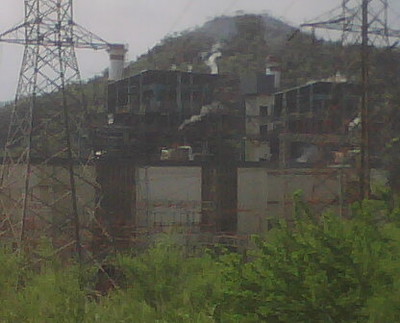The image depicts an eerie-looking power plant scene enveloped in an overcast and hazy atmosphere. This grainy, small square photo prominently features two tall towers resembling erector-set power line structures, positioned on each side of the plant. Below the towers, a thick layer of low trees and bushes covers about a third of the foreground, blending with the concrete guard wall of the power plant behind it. The plant itself is composed of perfectly square and rectangular multi-level buildings, with several tall smokestacks belching steam. In the background, a large hill or mountaintop covered in trees subtly looms over the scene. The sky above is a washed-out gray, appearing almost as one continuous cloud, adding to the chilling aura of the setting.